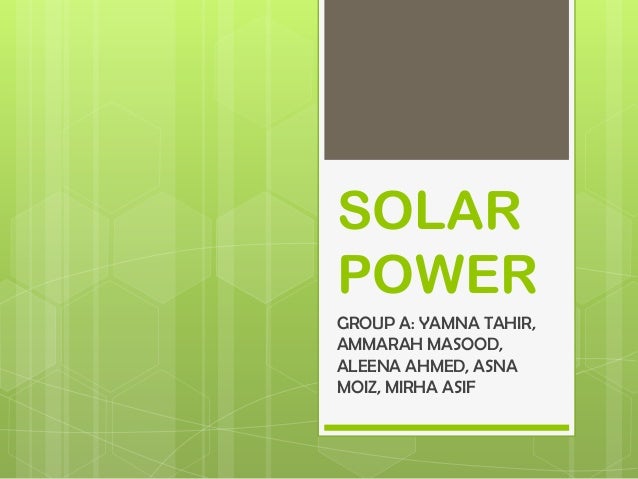The image shows the cover slide of a PowerPoint presentation, featuring a predominantly lime green background with various translucent geometric designs, including hexagons and criss-cross patterns. At the top center, there is a light brown rectangular design element. The focal point of the slide is a horizontally aligned white rectangle with a black square in its top section, creating thin vertical white borders. Within this rectangle, large green uppercase text reads "SOLAR POWER," followed by smaller black text that states "Group A: Yamna Tahir, Amara Masood, Alina Ahmed, Asna Moyes, and Mirha Asif." The overall aesthetic is modern and visually engaging, with the green background and layered semi-opaque patterns giving it a dynamic and contemporary feel.